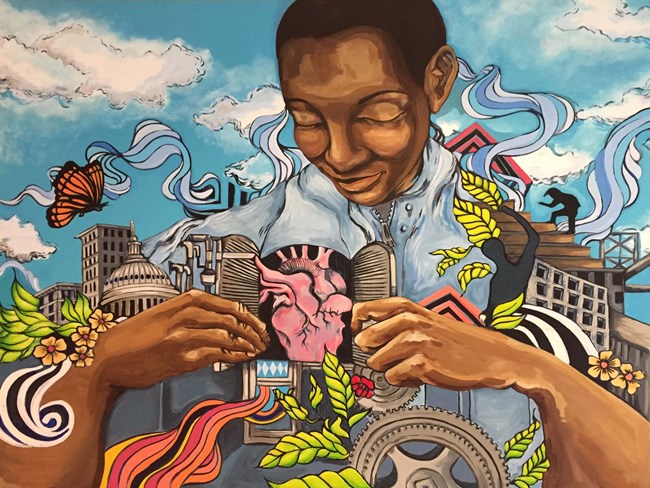The image is a highly detailed and vivid mural-style drawing, resembling a large wall painting. At the center of the piece is a dark-skinned man, possibly African American or Indian, with very short hair. He is prominently depicted wearing a blue zippered vest, and the primary focus is on his chest, which he is opening with his hands like doors to reveal a pink cartoon heart inside. The man is looking down at the heart with a gentle smile.

In the background, the sky is a brilliant blue filled with fluffy white clouds. There are several monarch butterflies fluttering around. Behind the man, architectural elements feature prominently, including what appears to be the Capitol Building alongside other tall structures. A shadowy figure of a man climbing steps is also visible.

The illustration is lush with additional details such as green branches, flowers, leaves, gears, and screws scattered throughout the image. Whimsical elements like waves and ribbon swirls float around the man, enhancing the dreamy and intricate nature of the mural. The overall effect is a rich tapestry of various symbols, all centered around the theme of unveiling and exploring the heart.